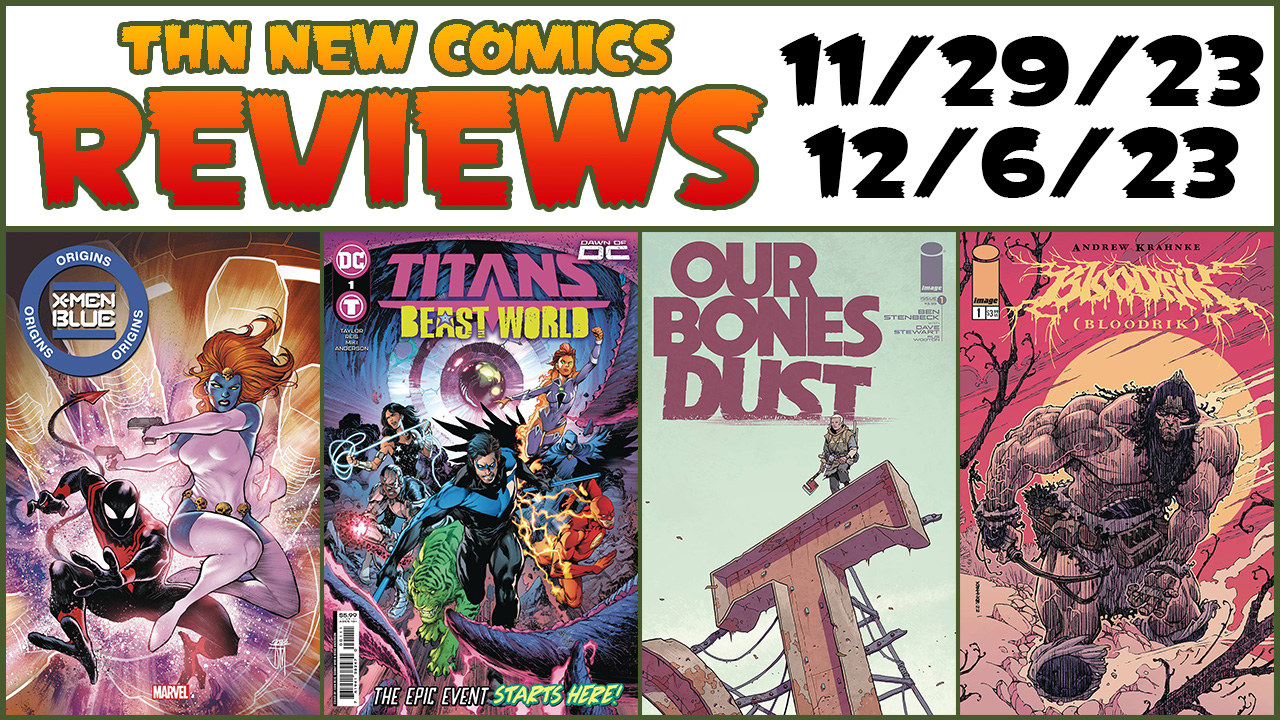This image is a horizontal advertisement for comic books, prominently labeled with the heading "THN New Comics Reviews" and the dates "11-29-23" and "12-6-23" in thick black ink against a white background. Below the heading, there are four vibrant and colorful comic book covers.

1. The first cover features "X-Men Blue," showcasing Marvel superheroes including a figure dressed in an all-black and red costume along with a woman, bursting through the page.
   
2. The second cover is for the "Titans," titled "Beast World," depicting superheroes in black and blue costumes flying through the air.

3. The third comic, labeled "Our Bones Dust," shows a man standing on what appears to be a construction site, against a light blue background with dusty rose lettering.

4. The last cover is more difficult to read due to distorted letters but features a gigantic, muscular monster-like figure, almost resembling a colossal gorilla.

All backgrounds are brightly colored, typical of comic book art, with shades of red, yellow, orange, blue, and some paler tones for variety. The advertisement is visually striking, aimed at promoting the latest comic book releases.